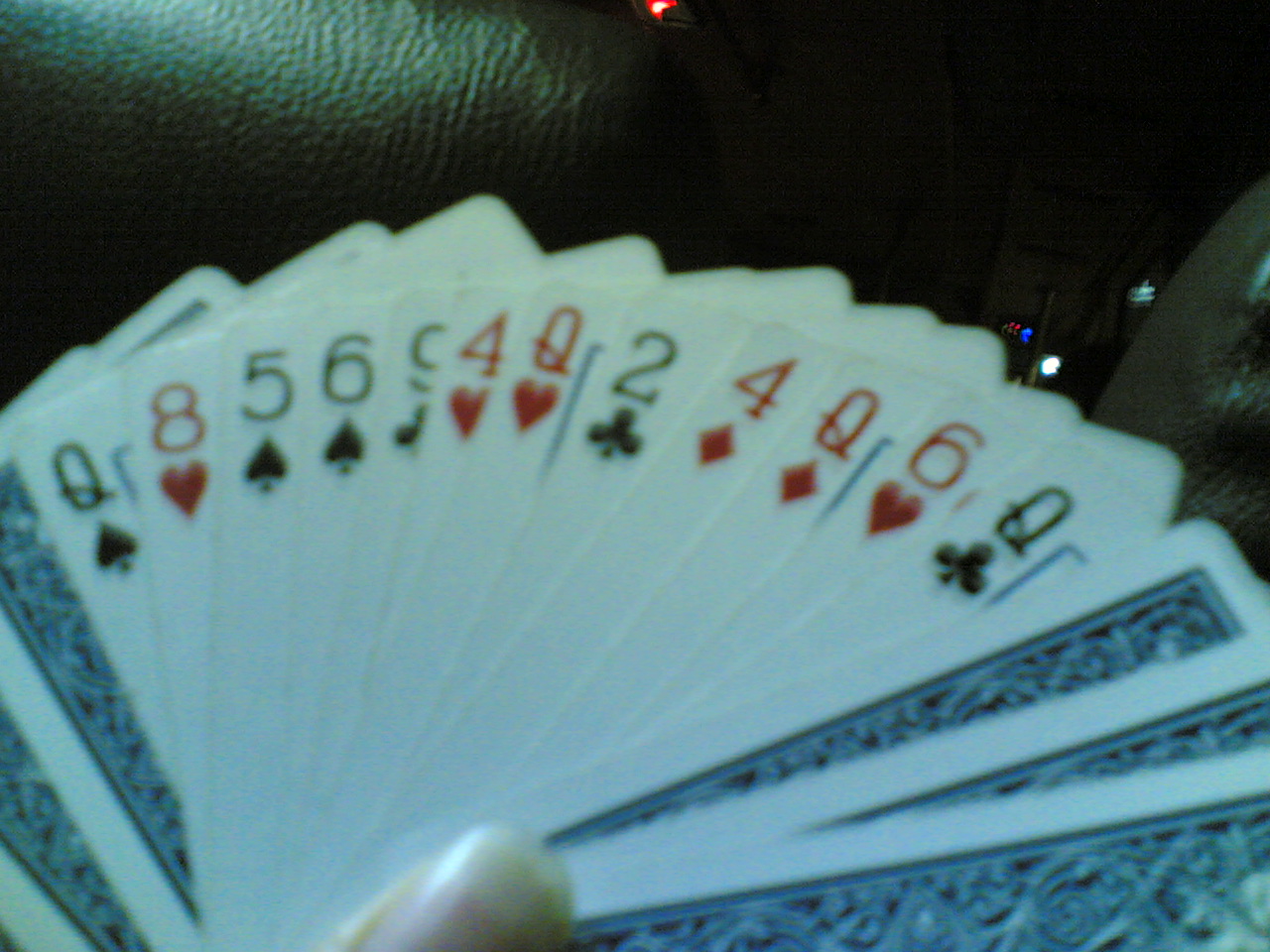A close-up image captures a deck of cards being fanned out, sharply showcasing the intricate details of each card's number and suit. The cards are held delicately, with only the thumb's fingernail visible, suggesting the careful, precise movement of the holder. In the background, the textured grain of a leather seat is evident, implying the setting is inside a vehicle. Further adding to this impression, a lit car dashboard can be seen in the distance, glowing softly against the darkness of the car's interior. Among the cards displayed, specific ones stand out, including the queen of spades, eight of hearts, five of spades, six of spades, four of hearts, queen of hearts, two of clubs, and four of diamonds. The arrangement offers a glimpse into a moment of casual gameplay or a demonstration of card handling within the intimate confines of a vehicle.